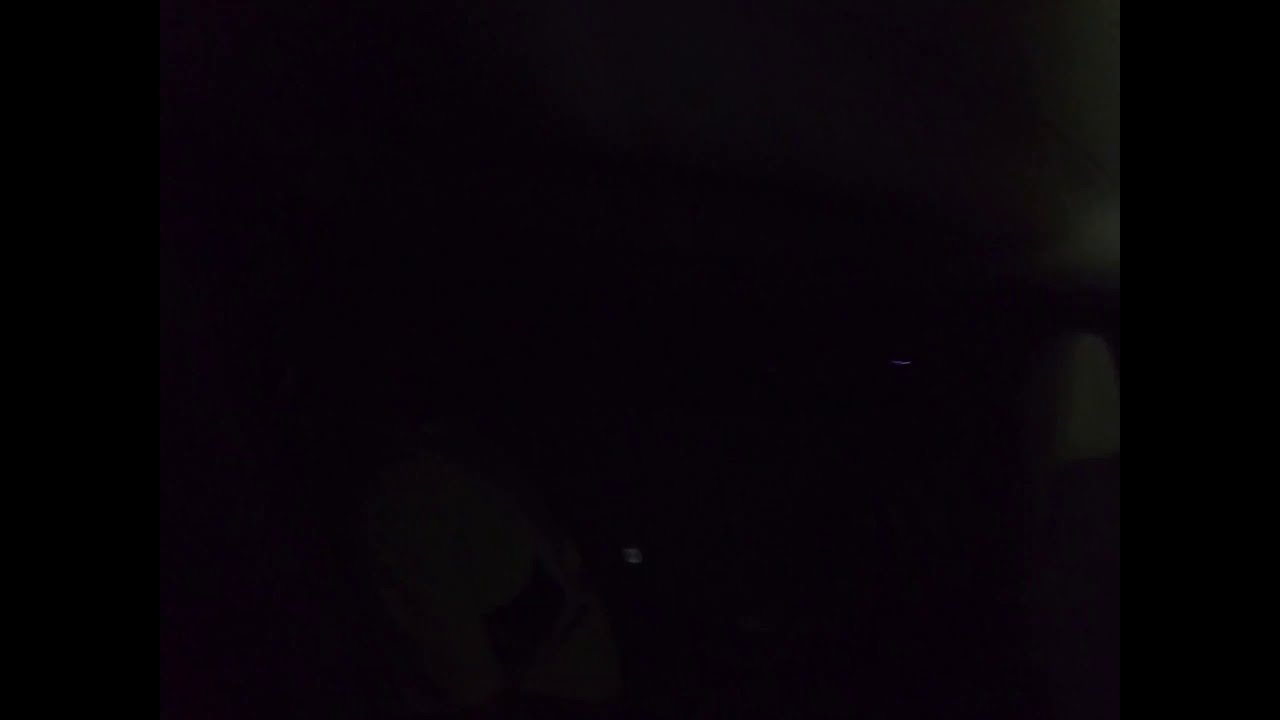The image is predominantly a very, very dark rectangle where discerning specific details is extremely difficult. The overall appearance is almost entirely black, with minimal variation. Along the right side, spanning from top to bottom, there is a black bar that is slightly distinguishable. Towards the left third of the image, there are subtle shadings that appear slightly lighter, almost a shade of dark gray. On the bottom left, and just to the left of the right black bar, there are faint patches of purple and dark green. Near the bottom center of the picture, a small, blurry reddish or pink line is visible beside a slightly lit area. Despite these minor differences in color and shading, the image essentially remains a solid black rectangle, with no clear objects or distinguishing features discernible due to the pervasive darkness.